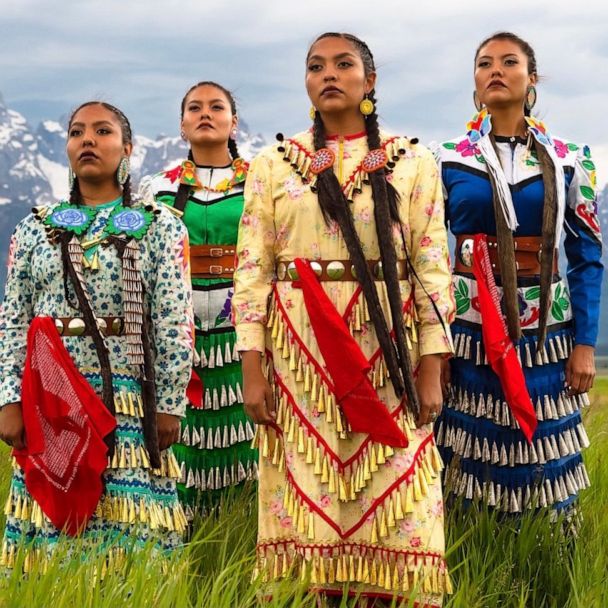In this vibrant and evocative image, four Native American women stand in a field of deep green grass, their stoic gazes fixed into the distance. Each woman is adorned in an ornate, traditional dress that showcases a tapestry of colors and intricate designs. One wears a yellow floral dress adorned with red and yellow tassels, another a solid blue dress with embroidered or appliqued flowers and white tassels, the third dons a green dress paired with white tassels, and the fourth features a teal skirt with white tassels and a white top decorated with teal flowers.

Their long hair is intricately braided in pigtails, and they each wear large earrings and have red bandanas hanging from belts adorned with medallions. The image, taken from a low angle, emphasizes their proud postures and cultural attire. The background reveals a sweeping mountainous landscape with snow-capped peaks under a cloudy sky. This powerful photograph captures both the beauty and the cultural heritage of these Indigenous women.